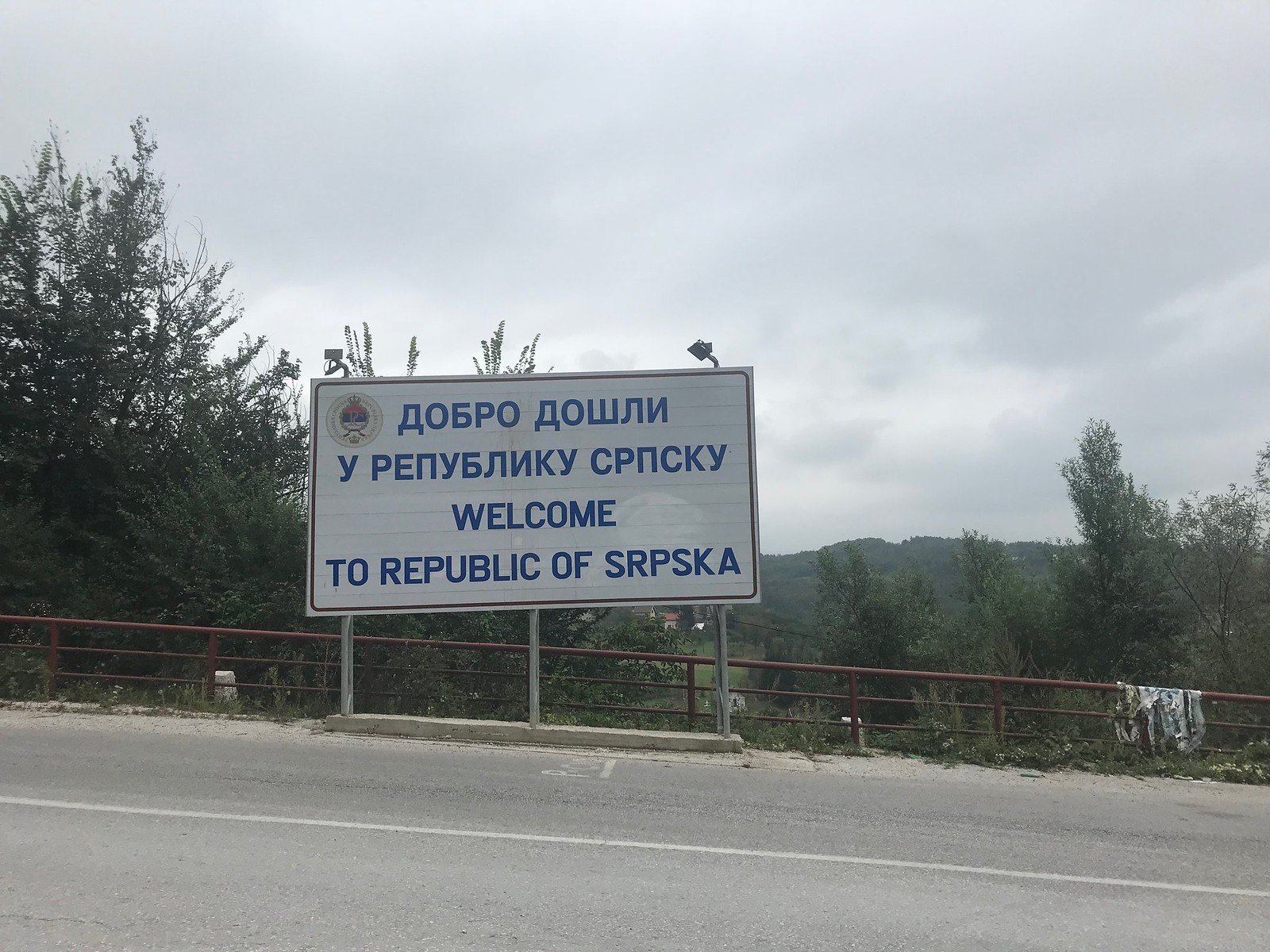This image features a roadside sign on a concrete road at a higher elevation, giving a vantage point that looks down into a valley. The backdrop includes brown metal guardrails and a landscape of distant, low-lying hills and forested areas. The sky is overcast and filled with gray, rain-threatening clouds. Centered in the photo, the white billboard displays blue text with the top part in Cyrillic and an English translation below, which reads "Welcome to Republic of Srpska." The sign also bears a crest in the top left corner, featuring red, blue, and white stripes with the letter "R" and a small crown.